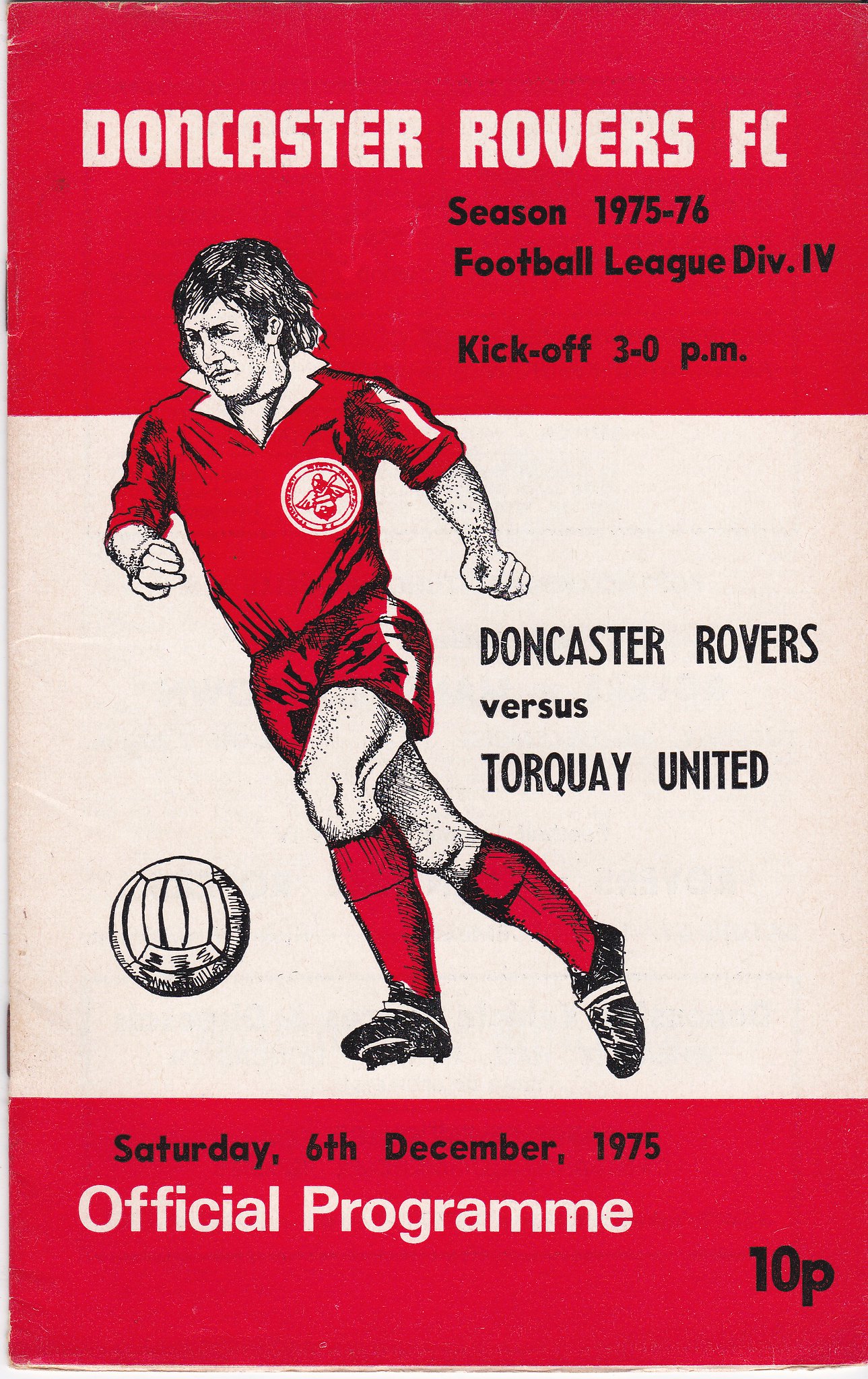The cover image features a football program for the Doncaster Rovers FC. The cover is divided into three horizontal bands—red at the top, white in the middle, and red at the bottom. At the top, in a white font, it reads "Doncaster Rovers FC," followed by "Season 1975-76 Football League Div. 4 Kickoff 3:00 p.m." in black against the red background. The middle band has a white background with a drawn image of a footballer in motion. The player is depicted with black hair, wearing a red shirt, white shorts with a red stripe, red socks, and black cleats, with a white ball in front of him. Flanking the image, the text "Doncaster Rovers versus Torquay United" is displayed in black. The bottom band, similar to the top, is solid red and features the text "Saturday 6th December 1975 Official Program" in white, with "10p" in black. The design and layout indicate it is the official program for the match.